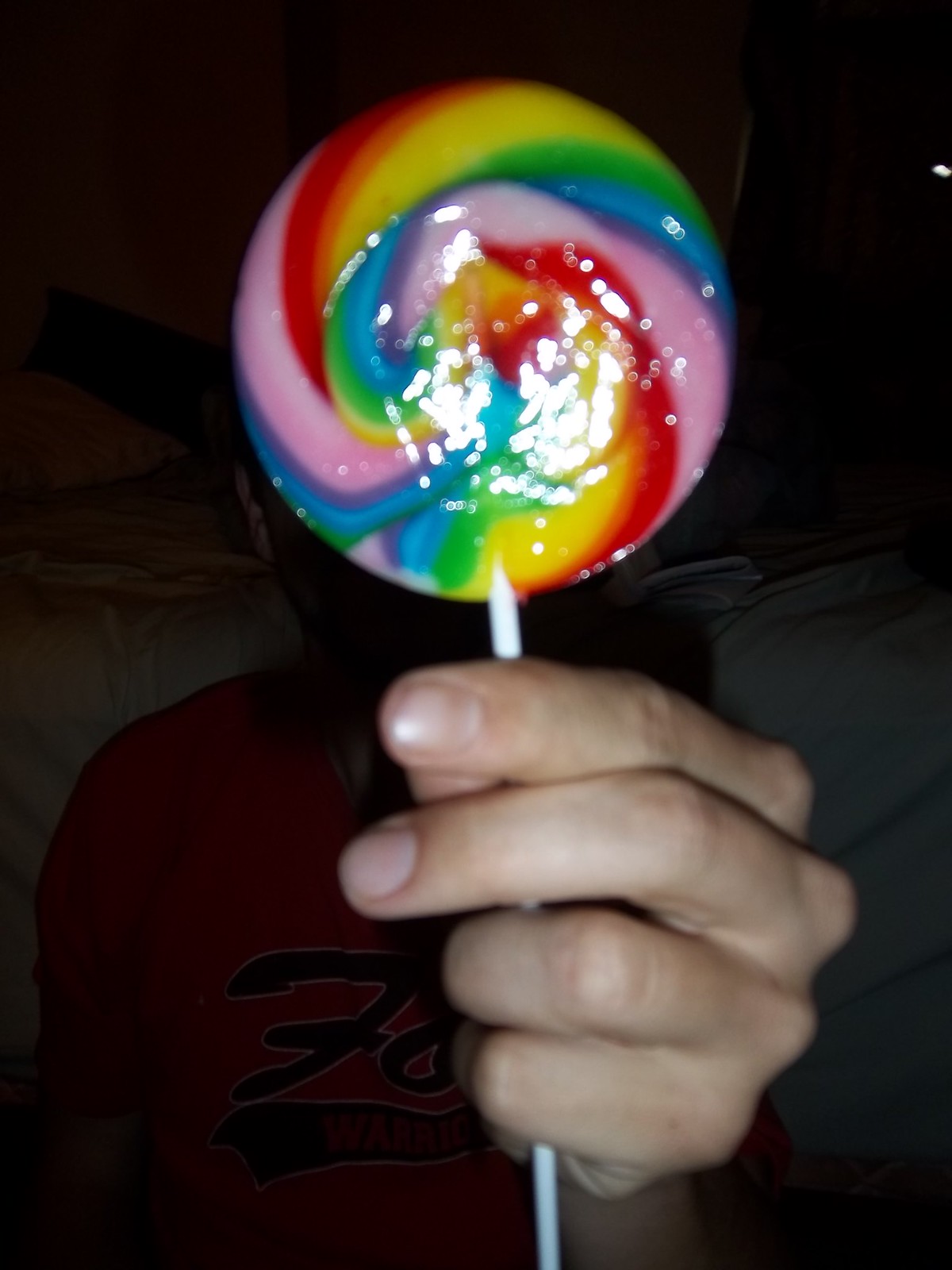In this close-up photograph, a hand is holding a rainbow-colored, swirled lollipop with a white stick. The lollipop appears very shiny, reflecting the camera flash, and slightly blurry as if the image is out of focus. The background is notably dark, emphasizing the lollipop as the focal point, with hints of a bed with white sheets and a wall behind. The hand, which has unpainted fingernails suggesting it might belong to a female, is positioned with the thumb and two first fingers extended outwards and the lower ring and pinky fingers grasping the stick. The individual, whose face is obscured by the lollipop, is wearing a red t-shirt with a black-lettered 'F' prominently displayed, possibly alongside other letters or symbols that are partially obscured. The scene suggests the person might be sitting on the floor in front of an unmade bed.